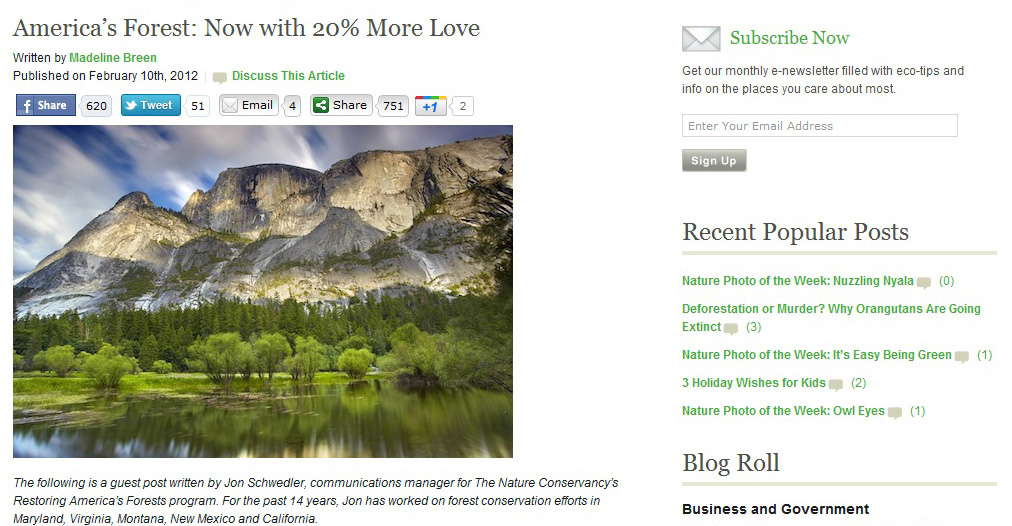**Detailed Caption:**

The image is a detailed screenshot of a digital newsletter featuring an article titled "America's Forest, Now with 20% More Love," written by Madeleine Breen and published on February 10, 2012. The layout is divided into two main sections: the left side contains the article, and the right side provides information about the newsletter.

On the left, at the top of the article, there's a set of social media icons for sharing the content via Facebook, Twitter, and email, along with engagement metrics displaying "7.51," "+1," and "2." Beneath these icons, there's a picturesque photo showcasing a serene mountainscape with wispy clouds, blue skies, and a lush forested river valley. The caption for this image reads: "The following is a guest post written by John Schwedler, Communications Manager for the Nature Conservancy's Restoring America's Forests Program. For the past 14 years, John has worked on forest conservation efforts in Maryland, Virginia, Montana, New Mexico, and California."

On the right side, the newsletter information is prominent, starting with a call-to-action reading, "Subscribe Now: Get our monthly e-newsletter filled with eco-tips and info on the places you care about most," followed by a field to enter an email address for subscription. Below this subscription section, there's a list of headings under "Recent Popular Posts," featuring topics such as "Nature Photo of the Week," "Deforestation or Murder," "Three Holiday Wishes for Kids," "Blog Role," and "Business and Government."

This screenshot encapsulates a harmonious blend of engaging content and useful information, encouraging readers to explore and subscribe for more eco-friendly news and tips.